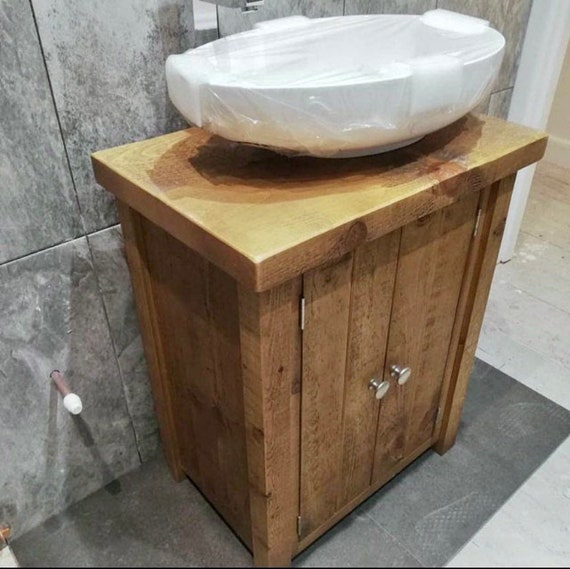This photograph showcases a bathroom sink under construction. The setting features a medium-colored wooden cabinet with silver knobs and two hinged doors on the front. Above the cabinet is a rustic wooden countertop holding an oval-shaped white ceramic basin, which is wrapped in clear plastic and protected by pieces of styrofoam. The surrounding environment includes a gray floor with dark gray tiles directly beneath the cabinet, transitioning to a lighter gray area that might resemble marble. The gray wall behind the cabinet displays a small capped valve near the bottom left, suggesting its future connection to the sink. Adjacent to the cabinet, a door stopper with a white tip is visible. The cabinet is positioned slightly at an angle, with the left side facing the camera more directly. The scene appears to be either a real-life household bathroom setup in mid-renovation or a display area for bathroom fixtures.